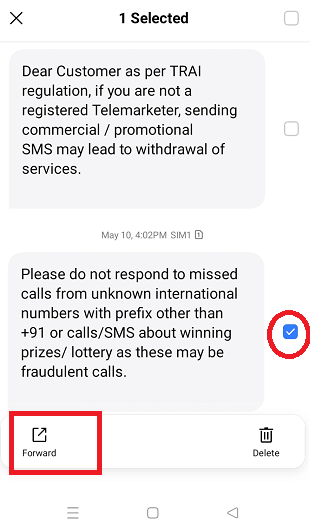A rectangular screenshot of a messaging screen is displayed, featuring a predominantly white background. In the upper left corner, a black 'X' icon is present for closing the screen. Centralized at the top, the bold black text reads, "One Selected," indicating a selected item within the interface. To the right of this text, there is a gray-outlined, unchecked checkbox with a white interior. Below this top section, a gray horizontal bar runs across the screen, separating these elements from the messages below.

The message section contains multiple entries displayed in rectangular, light gray boxes, each holding black text. Notably, on the right side of the third message, a checkmark box is highlighted with a red marker. This box is checked, showing a blue background and a white checkmark in its center. Additionally, an icon marked with a red rectangular border indicates the forward button, accompanied by the word "Forward" below it.

Further down on the right side, there is another button labeled "Delete," featuring a trash icon above it. At the bottom of the screenshot, typical smartphone navigation buttons are visible: three light gray vertical lines for opening different windows on the left, a square-shaped home button in the center, and a triangular-shaped back button on the right. These elements collectively detail the interface and functionalities visible within the screenshot.